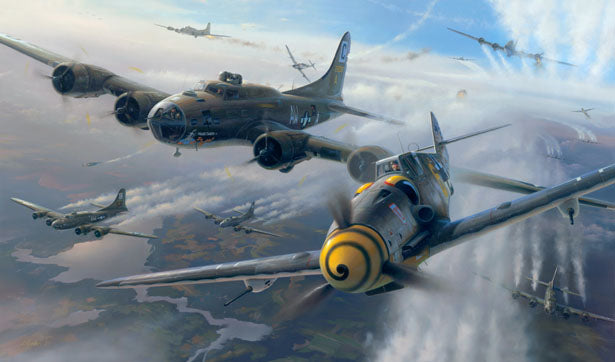The image, which appears to be a horizontal rectangle screenshot or artwork, depicts a vivid World War II aerial scene. Dominating the clear blue sky with patches of thin white clouds, a fleet of fighter jets and bombers fly in close formation at an angle toward the viewer. The planes, mostly dark gray or dark blue, have propellers at their front cylinders, with some featuring additional propellers along their wings. Prominently, the lead plane showcases a distinctive black-and-yellow swirly propeller design. Beneath the airborne spectacle, a patchwork landscape of dark blue and green earth is visible through the clouds, interspersed with a dark gray body of water. The scene evokes a sense of coordinated aerial might, with elements of smoke trailing from the engines, lending authenticity to the wartime atmosphere.